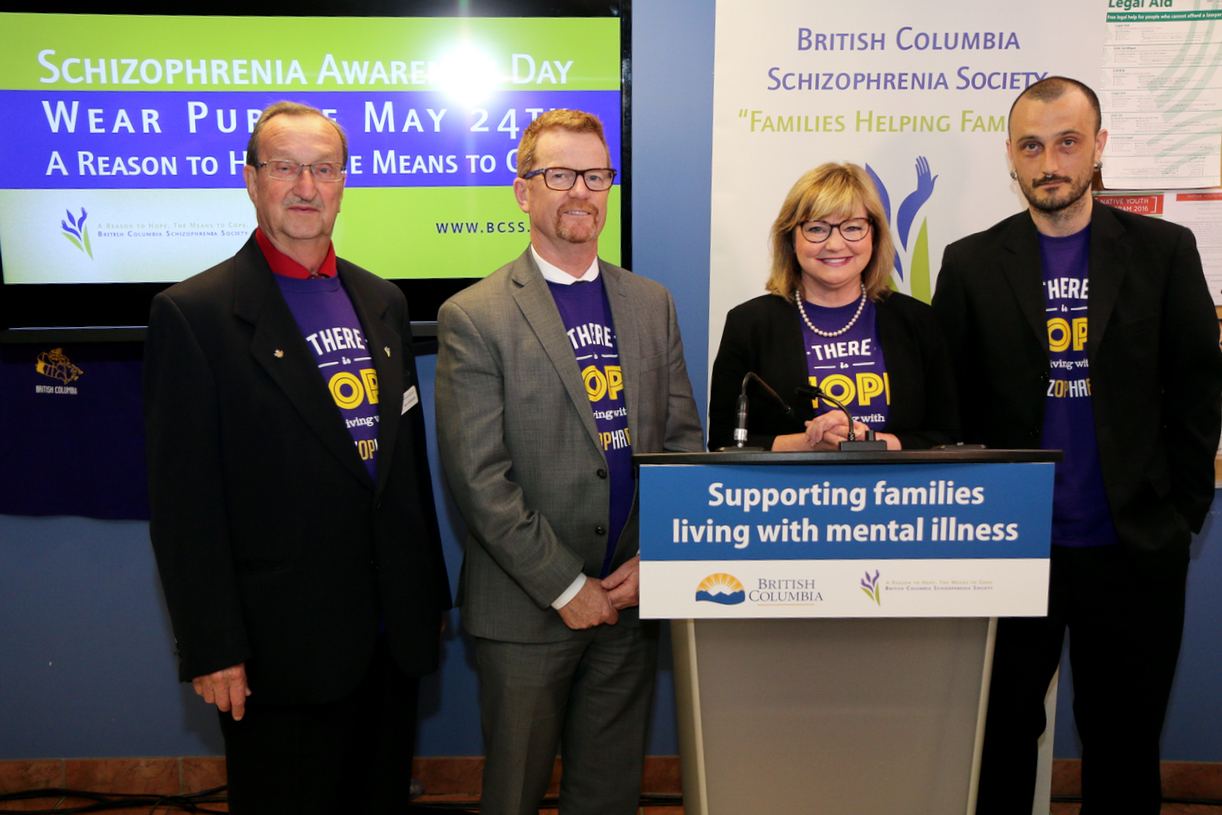The image depicts an indoor setting at a conference, featuring four speakers standing behind a podium. The group consists of three males and one female, all of varying ages and dressed in sports coats over blue t-shirts. Each shirt bears some white and yellow text, partially visible under their jackets. 

Starting from the left, the first man has short blonde hair, glasses, a mustache, and is wearing a black suit jacket. To his right is another man in a grey suit, with ginger hair, a small beard, a mustache, and glasses. The woman, positioned directly in front of the podium, has shoulder-length blonde hair, wears black glasses and a pearl necklace, and is dressed in a black suit jacket. The last man on the right is tall, with shaved dark hair, a mustache, and a beard, also wearing a black suit jacket.

The podium features a blue and white sign that reads "Supporting Families Living with Mental Illness." Behind the speakers, there's a TV screen displaying "Schizophrenia Awareness Day. Wear Purple May 24th." Additionally, another banner behind them reads, "British Columbia Schizophrenia Society, Families Helping Families."